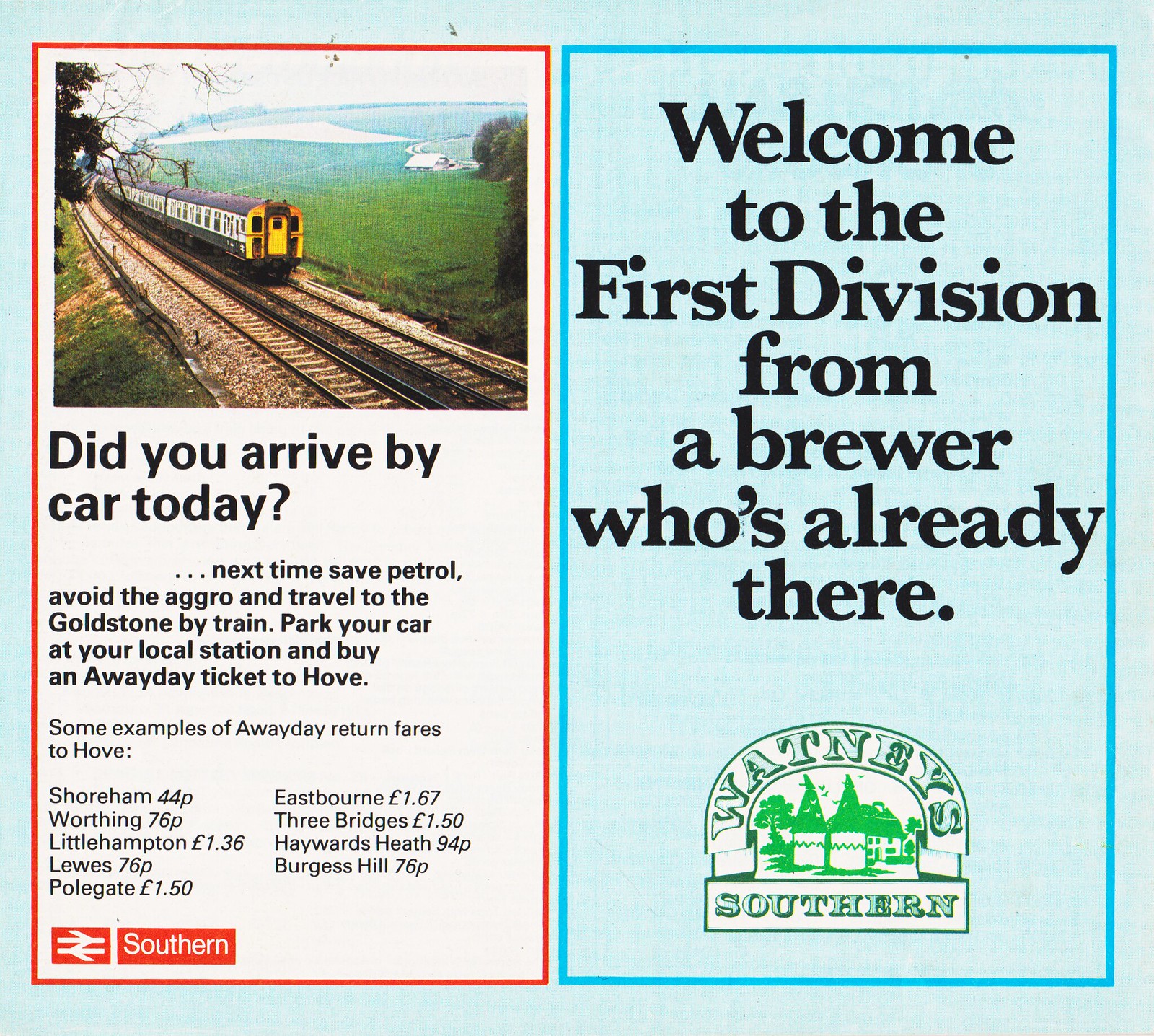This vintage British advertisement poster evokes a sense of nostalgia with its dual themed design. On the left side, a picturesque painting features a train traveling along a track surrounded by lush green landscapes and rolling mountains. Above this scenic image, a headline reads, "Did you arrive by car today?" followed by a suggestion to “save petrol, avoid the aggro, and travel to the Goldstone by train.” The ad encourages travelers to park their cars at local stations and purchase an away day ticket to Hove, listing example fares from various locations such as Shoreham (44p), Worthing (76p), Littlehampton (1.36 euros), and others. An emblem in the bottom left corner, colored in red with opposite-facing arrows, bears the word "Southern."

The right side of the poster, set against a light blue background with a darker blue border, carries a message for beer enthusiasts: "Welcome to the First Division, from a brewer who's already there." This text is center justified in black font above a green and white logo that reads "Watney Southern," featuring a castle motif. The colors used throughout the poster include black, white, gray, green, blue, yellow, and red, creating a vibrant and inviting advertisement.